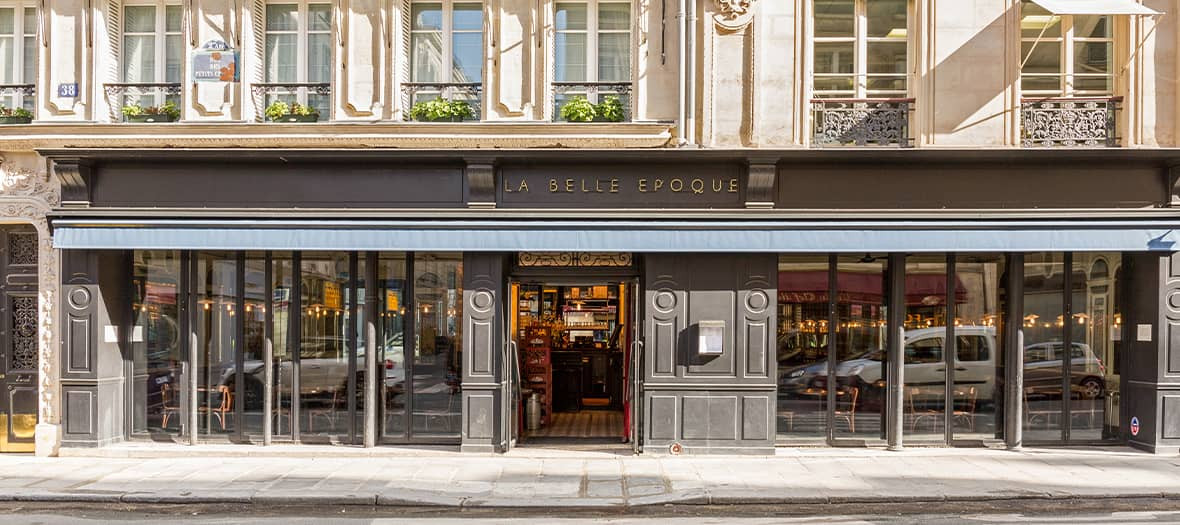This image showcases an outdoor view of LaBelle Epoque, a two-story building on a city street. The upper floor, tan and white in color, features multiple tall windows, each adorned with potted plants and enclosed by metal balcony railings, suggesting residential apartments or condos. The ground floor contrasts with a darker black and gray facade, dominated by large vertical glass windows that reflect the parked cars and the bustling street scene. Centrally positioned is a propped-open door beneath a brown sign displaying the name "LaBelle Epoque," inviting a glimpse into an interior space that reveals a bar area with lit candles, indicating a restaurant setting. The scene captures a serene moment with no visible people.